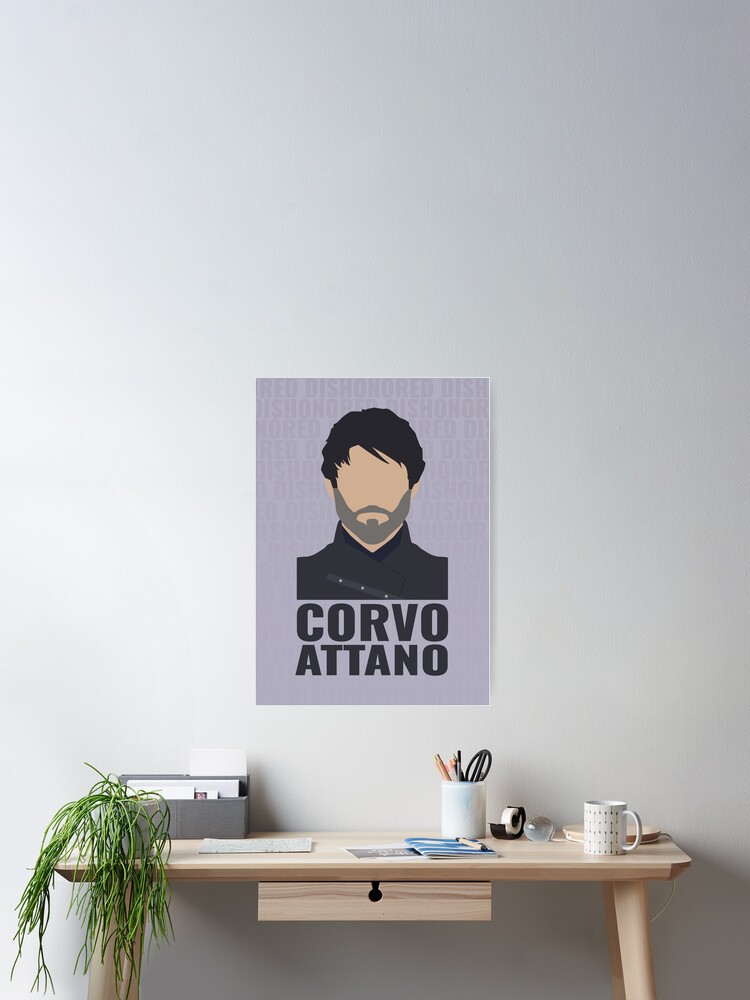The image is a vertically rectangular, full-color photograph taken indoors, featuring a small wooden desk positioned against an off-white wall. The lighting varies across the image, with the right side appearing darker, suggesting an artificial light source. On the left side of the desk, a cascading green plant adds a touch of nature. The desk is adorned with various items: a white coffee mug, a white desk lamp, a black tape dispenser, a white cup holding pens, pencils, and possibly a pair of scissors. A small drawer with a black keyhole is noticeable in the middle of the desk.

Above the desk hangs an artistic print, also vertically rectangular, depicting a faceless Caucasian male with black hair and a gray beard, dressed in a black shirt. The figure lacks eyes and a nose, creating a mysterious effect. Beneath the image, the name "Corvo Attano" is inscribed in bold, black capital letters.